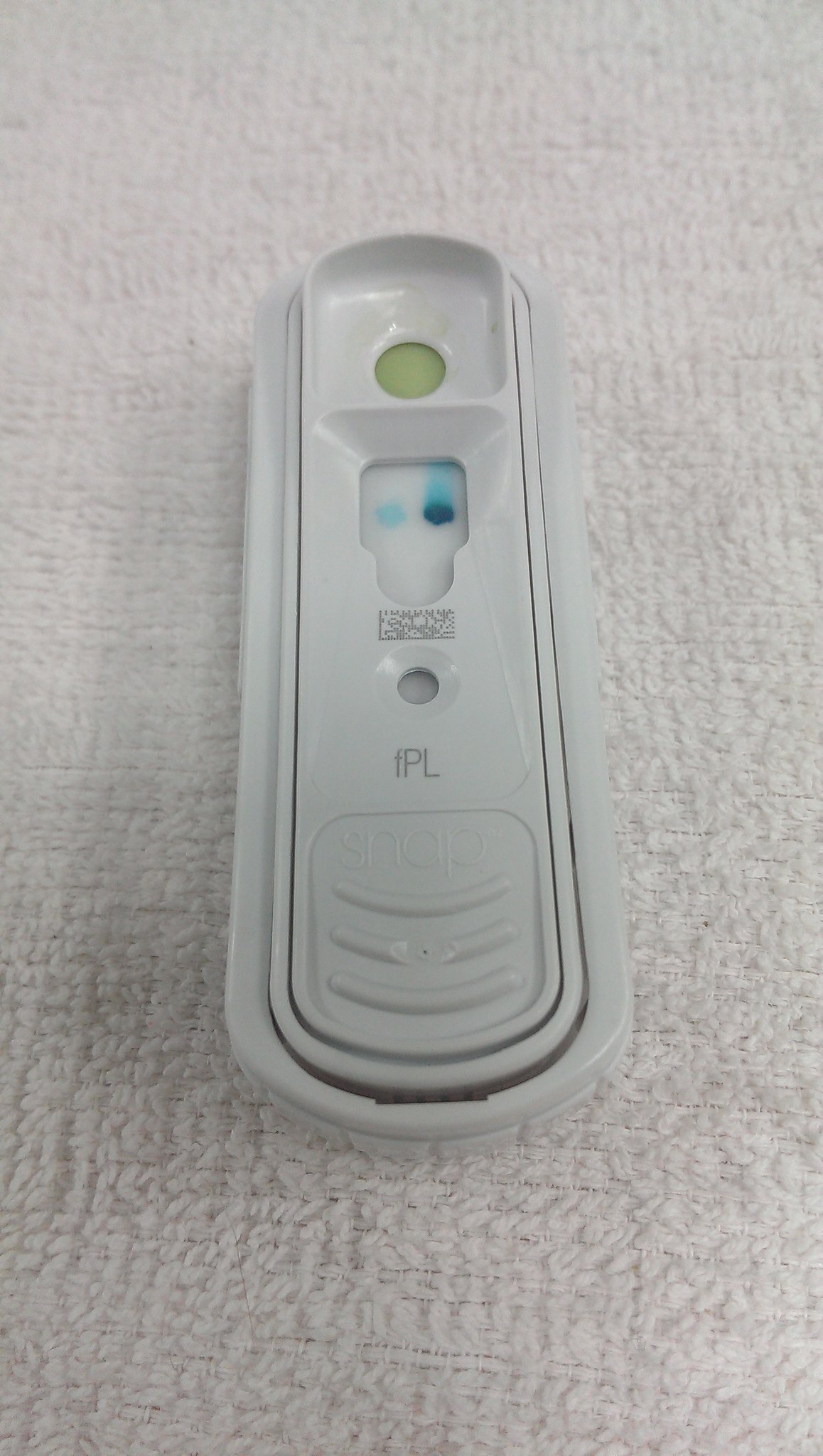This photograph depicts a rectangular, plastic test device, likely designed for medical or diagnostic purposes, such as a pregnancy or COVID-19 test. The white plastic casing is approximately a few inches long and an inch wide, featuring several distinct areas; a small circular hole, a moisture-wicking area with blue coloration, and another hole accompanied by raised, textured sections for handling. The device also contains the word "SNAP," suggesting a mechanism to activate or confirm the test results. The blue, water-colored trail within the wicking area could indicate a positive test result, similar to the visual cues used in COVID-19 tests, but it might also represent gender information, with blue possibly indicating a male. The test is placed on a woven white fabric, which helps to provide a sense of scale, confirming its compact size. The letters "FPL" are visible along with some unreadable text, further hinting at its specific use.